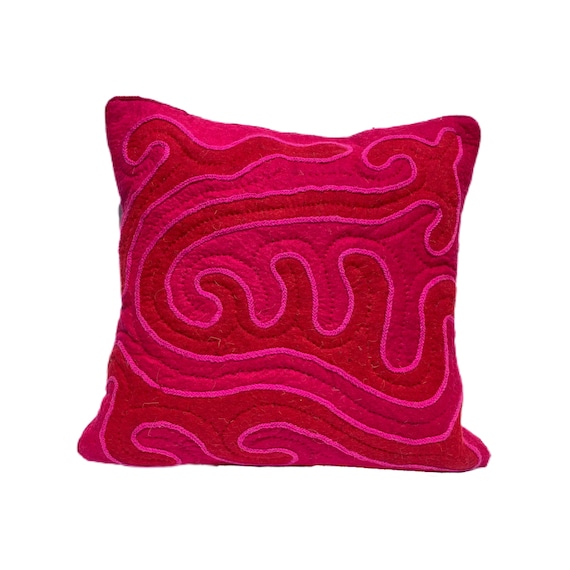This photograph showcases a brightly colored, square throw pillow with rounded corners, displayed on a flat, white surface in a minimalistic marketing style. The pillow features a striking abstract pattern of dark red and light pink wavy, serpentine lines that create an illusion of swirling motion. These lines originate from the upper right corner, curve around the center, and extend down to the lower right corner. The design is quilted, highlighted by subtle sewing lines that add texture to the surface. The combination of the vivid pink background and the dark red squiggles outlined in pink creates a visually appealing aesthetic. Overall, it's a standout decorative pillow, perfect for a couch.